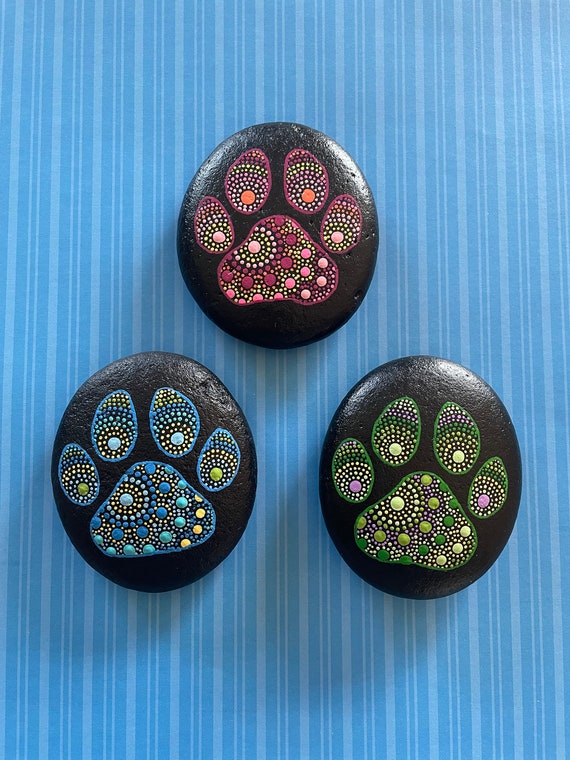The photograph features three black, oval-shaped stones adorned with intricate mosaic paw print designs, each crafted from small, colorful circular stones. Positioned on a vertically striped blue and light blue background, the image captures the upper stone with a vibrant paw print exhibiting shades of red, pink, orange, and yellow. Below, the stone on the bottom left showcases a design in varying hues of blue, teal, light green, and yellow, while the stone on the bottom right displays a paw print in a lush green, reminiscent of grass. The scene is brightly lit from the upper right, enhancing the decorative and meticulous detail of each unique paw print against the serene, wallpaper-like background.